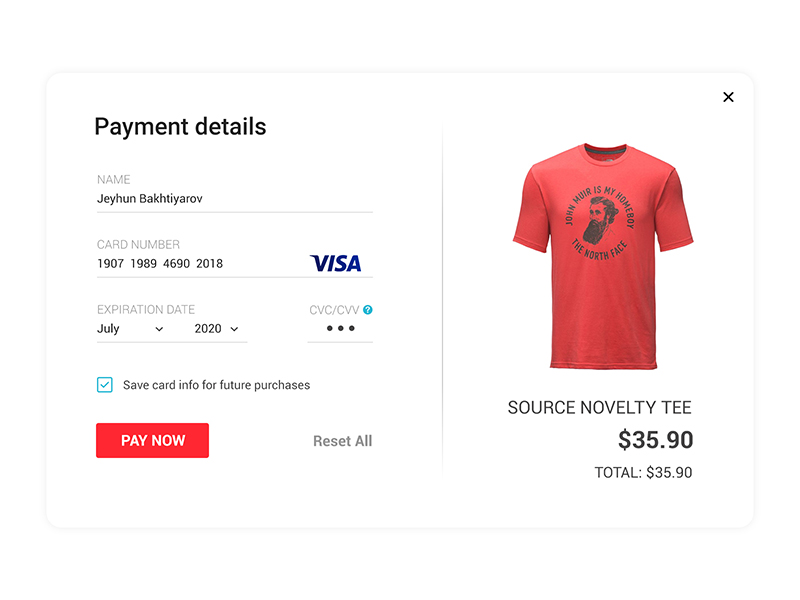The webpage from a clothing store is divided into two sections. 

On the left side, labeled "Payment Details" in large black text, various billing information fields are filled out. The "Name" field, in light gray text, displays "jhon.gov" in black text. Below that lies the "Card Number" field, which contains the number "1971 9894 6902 018." To its right, an icon indicates it is a Visa card. The "Expiration Date" field shows "July 2020," and the adjacent CVC-CVV field is masked with dots. Beneath these fields, a blue checkbox labeled "Save card for future purchases" is present. At the bottom, there is a prominent red button with "Pay Now" in white text, along with a gray button labeled "Reset All."

On the right side of the webpage is an image of a red short-sleeved shirt. The shirt features black text that reads "John Heard is my homeboy, The Northern Face," accompanied by a depiction of a man with long hair and a beard. Below the image is a price breakdown: "Source: Novelty Key, $35.90," with the total amount also listed as $35.90.